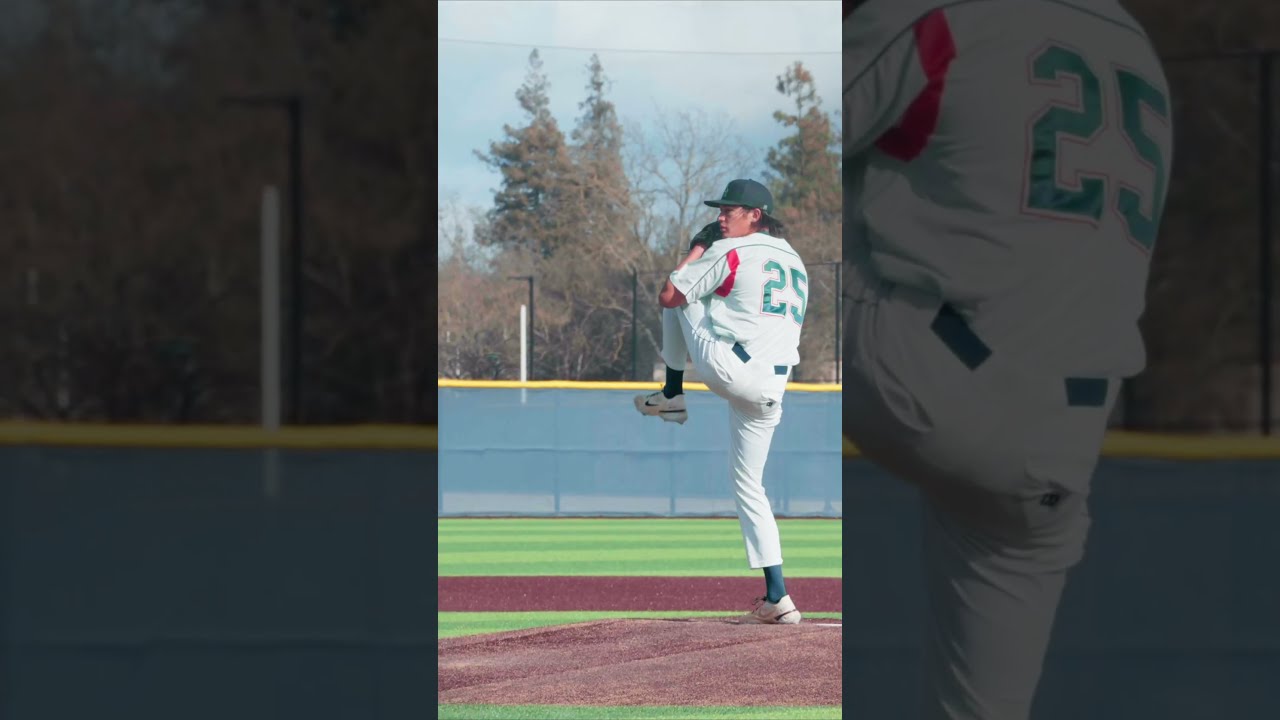In this image, we see a detailed shot of a baseball pitcher in full uniform, captured mid-windup on the pitcher's mound. The pitcher, sporting the number 25 on his back, is wearing a white uniform with one red stripe, white pants, and Nike cleats. His cap, dark blue or black, tops off his outfit. He stands on his right foot while his left leg is lifted high, knee level with his chest, and his arms are bent close to his face, preparing for the pitch. His profile is visible, facing left, suggesting he's of a slender build.

The setting features a distinct backdrop that includes a blue chain-link outfield fence with a yellow stripe on top, beyond which are green pine trees under a clear blue sky. This scene is essentially repeated and artistically enlarged to form the left and right side panels of the photograph, although these side panels are blurred or darkened for effect. The panel on the left is a close-up of the blue and yellow outfield wall, while the right panel presents a prominent close-up of the back of the pitcher’s uniform, clearly displaying the number 25. The central panel is the main focus, presenting the pitcher in sharp, high-definition detail, poised and ready to unleash his pitch.